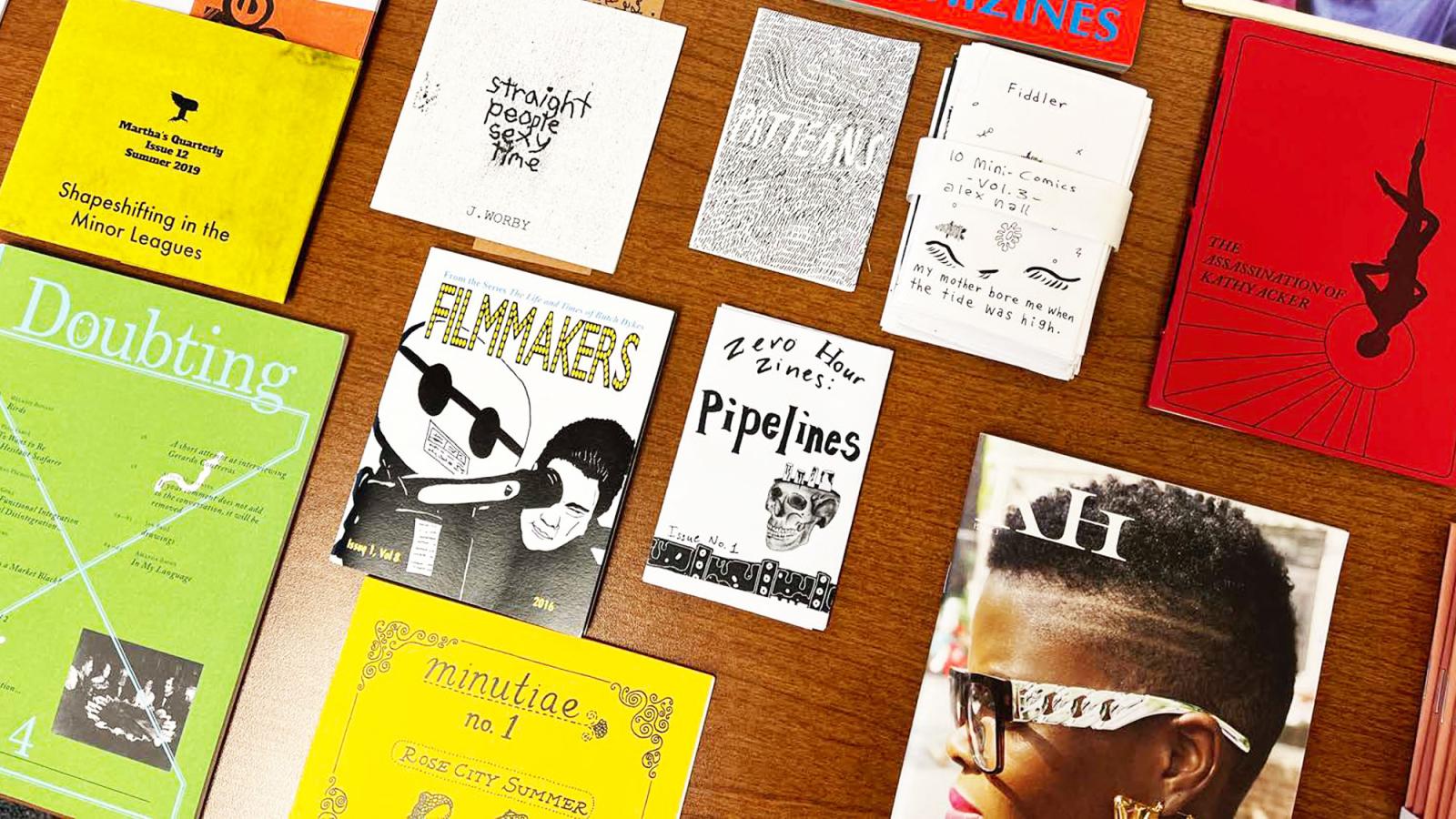On a glossy wooden table, there is an organized collection of various small press books, magazines, and pamphlets. The top right features a red-covered book titled "The Assassination of Kathy Acker," showcasing a figure hanging upside down in silhouette, evoking the imagery of the hanged man from tarot, set against a solar disk with radiating beams. Adjacent to it is "Fiddler, My Mother Bore Me When the Tide Was High," bundled among "10 Mini Comics, Volume 3" by Alex Nell. Following that is a book named "Patterns," distinguished by its crosshatched pencil drawing. Next is "Straight People Sexy Time" by Jay Werbe, presented with block writing. "Shapeshifting in the Minor Leagues" is another title contributing to the colorful assortment. 

In the second row, a green magazine titled "Doubting," presumably issue four, stands out with its list of articles. Nearby, two white rectangular pamphlets are displayed— "Filmmakers," featuring a black-and-white drawing of someone peering through a camera, and "Zero Hour Zines: Pipelines," which includes an intricate skull illustration. Below these is a yellow pamphlet labeled "Minutia number one, Rose City Summer." Completing the array is a magazine marked "KH," starring a black woman with striking black-framed glasses and bright red lipstick. Other publication covers are predominantly white, with notable exceptions including yellow and green.